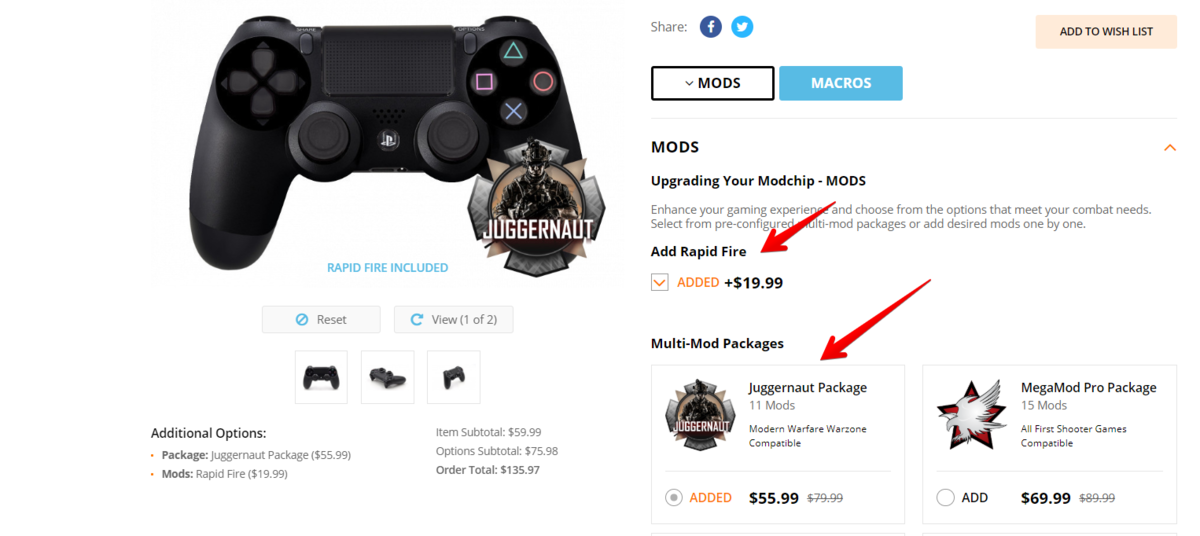Here we have a detailed look at a black PlayStation controller, designed with a familiar ergonomic style for those who have grown up playing on the PlayStation platform. The controller features two analog sticks positioned next to each handle for intuitive thumb control. The standard button layout includes a green triangle at the top, a red circle on the right, a blue X at the bottom, and a purple square on the left. Above the controller, the word "Juggernaut" is prominently displayed, although its exact significance is unclear, potentially indicating a special edition or a specific game-related brand. Nearby, various prompts suggest customizable options, like adding rapid fire capabilities or enhancing the overall package for an additional cost. This appears to be a promotional material or product listing aiming to highlight both the controller's versatile features and added functionalities for a more immersive gaming experience.